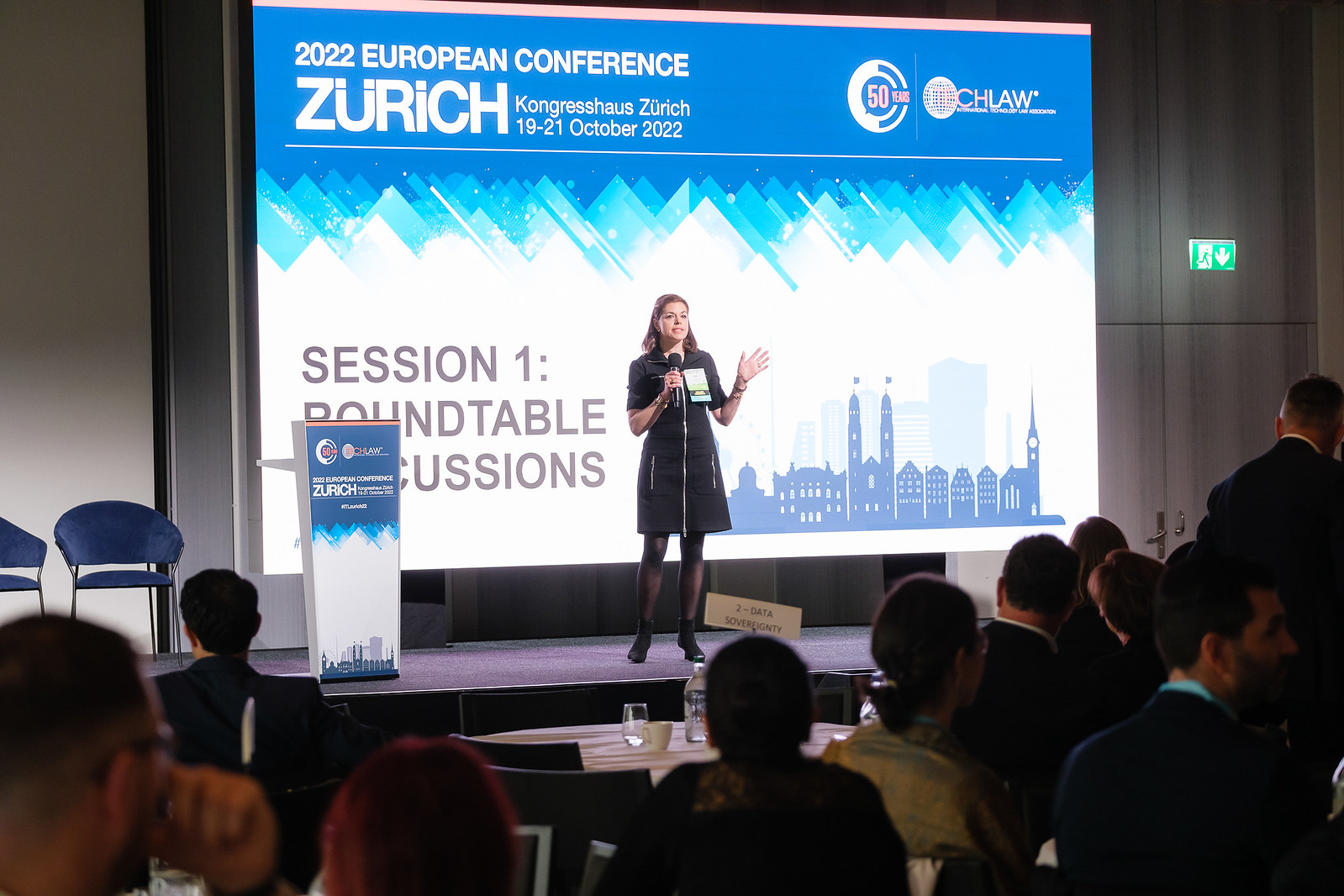In the image, a woman with shoulder-length brown hair stands on an elevated stage, holding a microphone near her face with her right hand and gesturing with her left. She is dressed in a black knee-length dress with a front zipper and silver-pocket accents, along with dark tights and dark boots. A fairly large membership tag hangs around her neck, suggesting she is at a conference or convention. Behind her, an illuminated projector screen displays information for the "2022 European Conference" held at Zurich Congress Haus, Zurich, from October 19 to 21, 2022. The backdrop features a blue background with abstract mountain shapes leading to a white lower half, and a blue silhouette of a city skyline on the bottom right. Text in white letters reads, "Session One Roundtable Discussions," accompanied by the logo "CHLAW" on the right. The stage has dark carpeting, and to the left of the woman stands a lectern with the same backdrop design. Two blue chairs are placed further to the left. In the foreground, an audience dressed in dark suits and fancy outfits sit at round tables equipped with water, glasses, and beverages, attentively listening to her presentation. A man stands on the far right side of the crowd, adding to the attentive atmosphere.